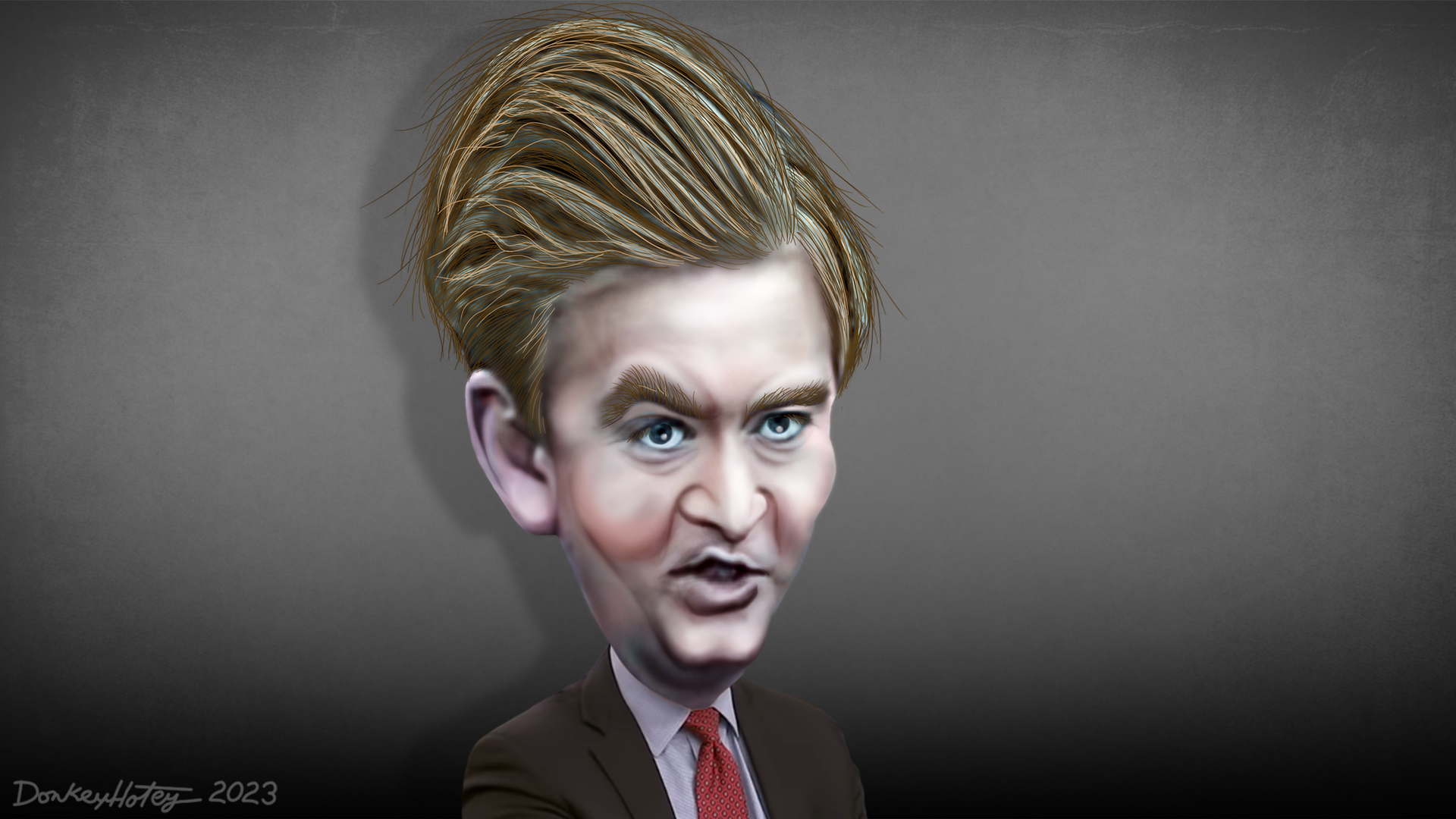This image is a distinct caricature of a famous Fox News reporter, featuring exaggerated elements and digitally drawn details. The character's brown hair, which dramatically rises about six inches high and sweeps to the left, stands out prominently. The hair detail is particularly noteworthy, massively higher than in real life. The character’s face is flesh-toned and slightly distorted, notably detailed with a single oversized ear in a pinkish-purple hue. Prominently displayed is the reporter’s raised right eyebrow, creating a questioning expression. His face tapers down to a double chin, contrasting with the thin chin mentioned in another description, highlighting the caricature’s artistic exaggeration.

The outfit consists of a brown sport coat paired with a violet-colored shirt, which another description notes as light blue, buttoned with a bold red and white polka-dotted tie. The facial features are further characterized by thick eyebrows, a pointed nose, and lips parted as if in mid-speech, adding to the contorted, expressive look. The background is a solid gray, and the lower left corner of the image bears the artist's signature, "Don Quixote 2023," affirming the artwork’s distinct style and creative liberties.